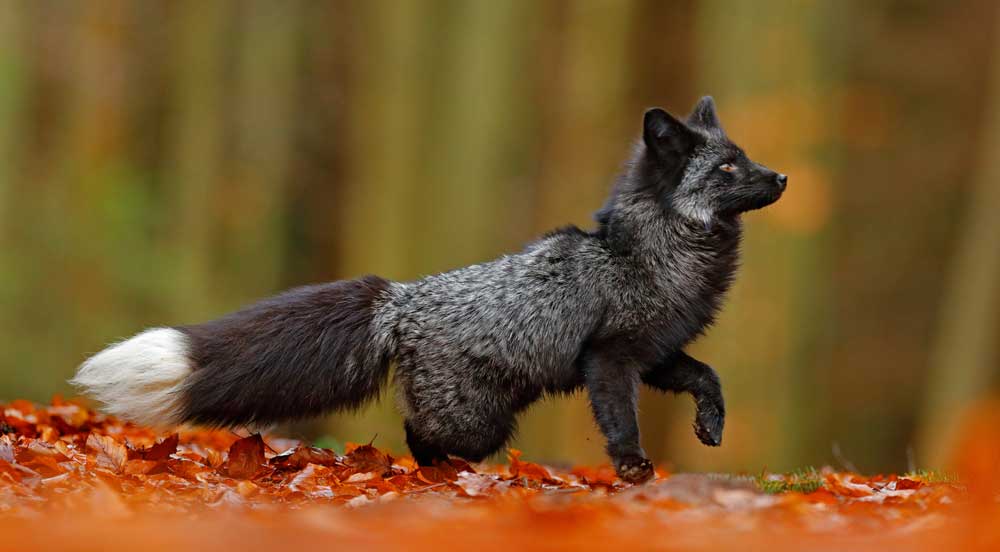The image captures a small, very tiny and cute black fox with dark gray fur and variegated splashes of white. Its body is almost completely black, including its solid black ears and predominantly black paws and legs. This fox has striking, glowing golden eyes and a very bushy tail that is nearly as long and thick as its body. The tail is distinctive with its brown coloring and a prominent white tip. The fox is prancing forward with its front left paw raised, as if about to move. It stands on a vibrant bed of red, orange, and yellow leaves, suggesting an autumn setting. The background is blurry but reveals green and brown tree trunks, indicating a forest environment filled with the rich colors of fall.